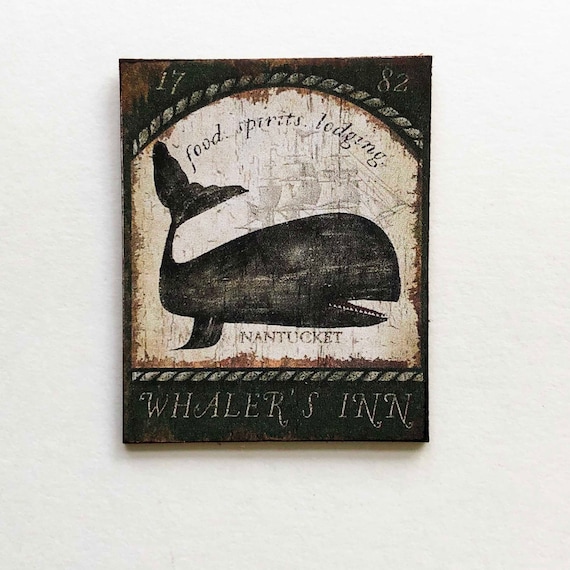This is a photograph of an antique advertising sign from 1782, likely for a historic pub or bar named Whalers Inn in Nantucket. The sign, which appears to be painted on wood, features a rustic and stylized depiction of a black whale with its mouth open and tail upward. The whale is centrally positioned, and behind it, faint images of a multi-masted sailing ship can be discerned, further evoking the whaling heritage.

At the top of the sign, "17" is painted on the left and "82" on the right, both within a black arch designed to resemble a rope. Below this, in block letters within a white central section, are the words "Food, Spirits, Lodging.” Directly beneath the whale in large, capitalized letters is the word "Nantucket." Toward the bottom of the sign, another rope-like design is depicted, and below this, the words "Whalers Inn" are written in white on a black background.

The sign features a color scheme dominated by blacks, whites, and tans, and appears to be mounted on a plain, off-white wall. The paint shows signs of age, with a crackled and slightly discolored finish, reinforcing its historical appearance.